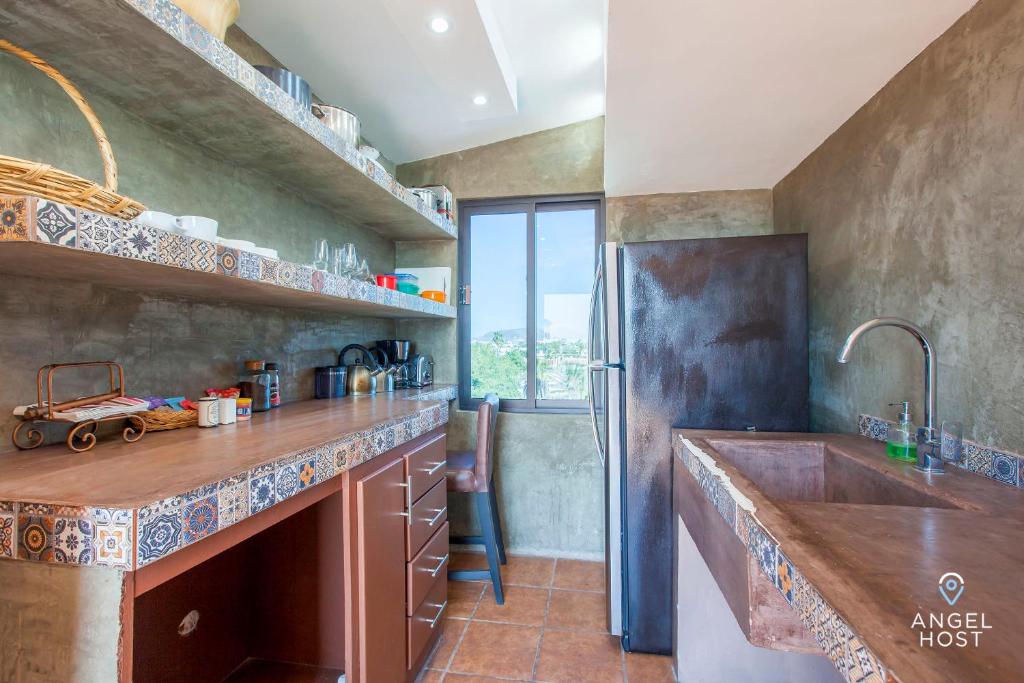This is a very detailed image of a narrow kitchen, evocative of a space in a motorhome but likely situated in a small house. The kitchen features a cozy setup with an intimate proximity to all elements. The countertops appear to be a brownish marble or stone, and the edges are adorned with a Mexican or Aztec-inspired mosaic tile trim, showcasing a mix of blue, yellow, and brown patterns.

Straight ahead, there's a window trimmed in gray, providing a view of trees and a building in the background. The walls around the window are painted in a light beige, complementing the overall warmth of the room. Below the window lies a large kitchen sink with a prominent silver faucet, flanked by green hand soap and a squirt bottle.

On the right side of the kitchen stands a black refrigerator, while towards the foreground sits a countertop possibly made of butcher block wood, adorned with decorative canisters, a salt and pepper shaker in white, and a filigree napkin holder. A chair at the end of this counter matches the copper color of the below-cabinetry and boasts gray wooden legs. 

The left side features shelves hosting a variety of glassware, mugs, and pottery. The upper shelf, near the ceiling, contains metallic pots, while the lower shelf displays a woven basket and various cups and glasses. Below these shelves on the counter are items like a salt shaker, baskets, and seasonings. 

In terms of appliances, there is no visible stove or oven, but a coffee pot and toaster are present on the counter. The flooring consists of large brown Mexican tiles, and the white drop ceiling integrates built-in lighting, enhancing the kitchen's overall illumination.

This richly adorned and space-efficient kitchen reflects a blend of practicality and artistic flair within a compact setting.